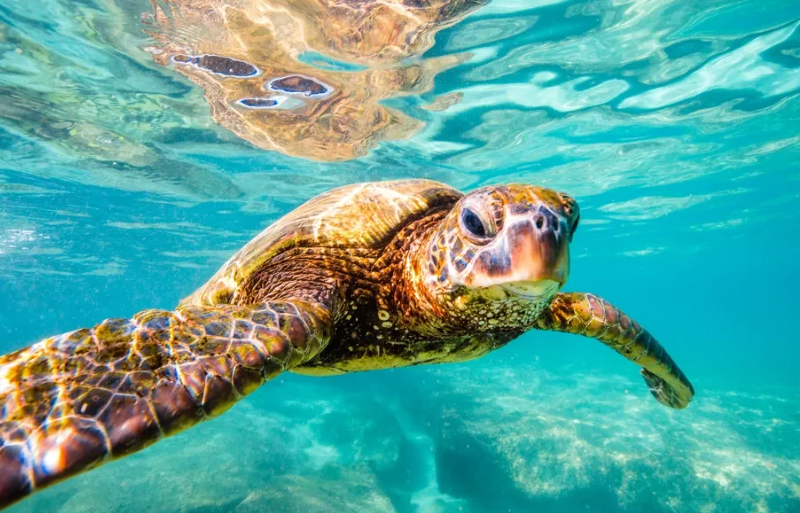This vivid, underwater photograph captures a close-up of a large loggerhead sea turtle swimming in clear, turquoise water. The realistic, horizontally-oriented image beautifully showcases the turtle's detailed features, including its expressive face with a slightly grouchy look and its distinctive yellow, white, black, and brown coloration. The turtle is centrally positioned, appearing almost to touch the lens with its outstretched flippers. The clear reflection of the turtle on the water's surface and the rocky ocean floor below add depth to the scene, highlighting the shallowness and clarity of the aquamarine water. The overall impression is one of serene solitude, with the majestic turtle as the sole subject in this mesmerizing aquatic environment.